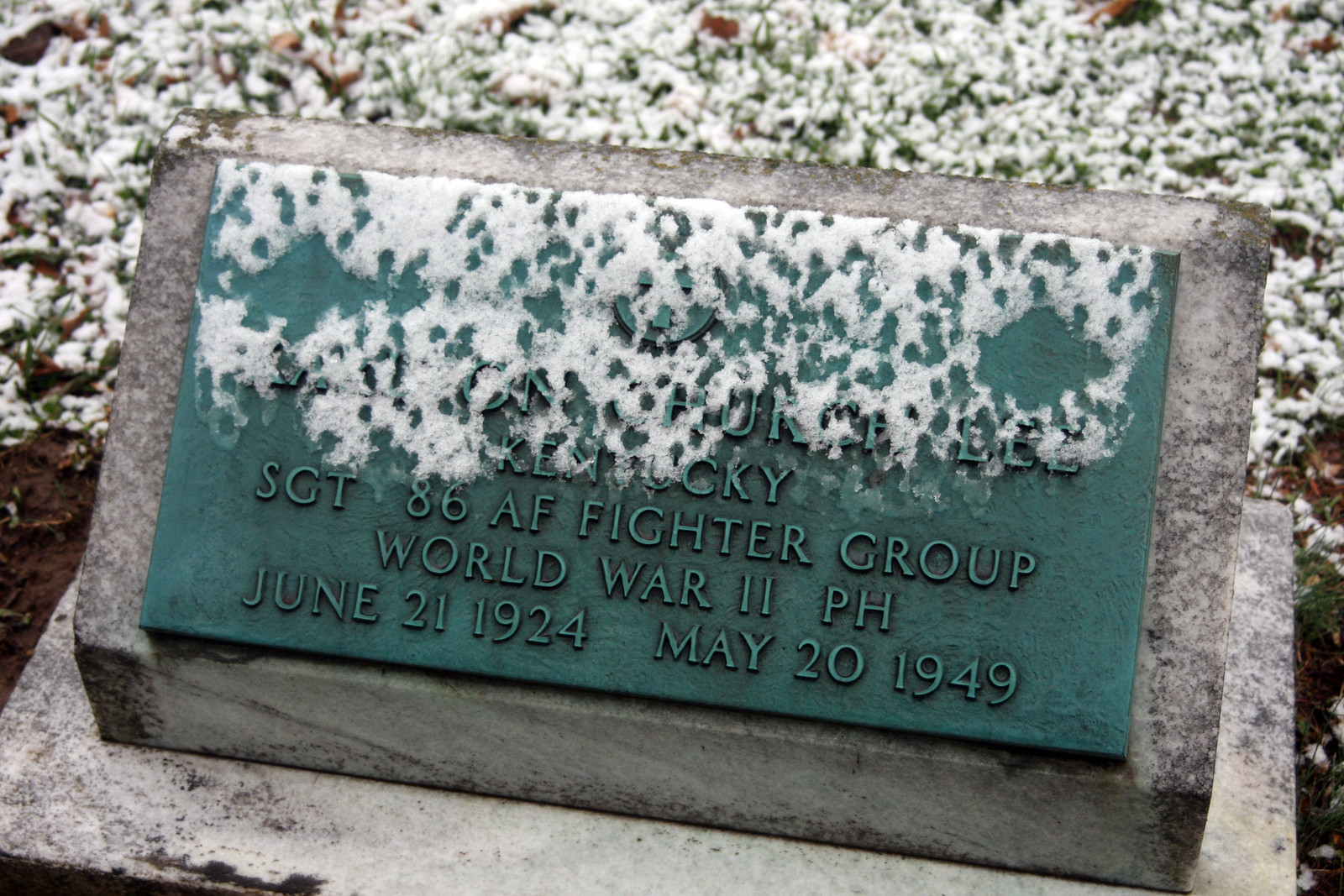This photograph captures a gravestone in a snowy cemetery. The prominently featured element is a teal-colored plaque affixed to a white and gray stone, which itself rests on another similar stone. Snow partially obscures the text on the plaque, which reads: "Ken Rocky, Sergeant, 86 AF Fighter Group, World War II, pH, June 21, 1924 - May 20, 1949." The surrounding area is covered in a layer of snow or icy frost, with patches of grass faintly visible through it.